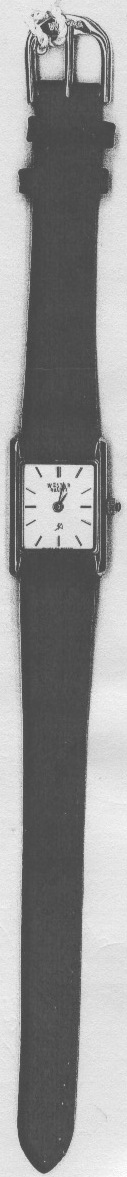This black-and-white photograph, presented in a long rectangular format with a white background, showcases an old-fashioned ladies' wristwatch suspended from the top by two thick threads. The watch features a silver horseshoe-shaped buckle at the top, followed by two dark-colored, likely black, straps that appear to be made of rubber. The square watch face is encased in a black frame, with silver details adorning its exterior.

The watch face itself is white, displaying hours marked by small black lines instead of traditional numbers. The hands of the watch are also black, distinctly pointing to 1 o'clock. Additionally, there is an illegible brand name printed underneath the number 12 on the dial. A small side knob or dial, situated on the right side of the watch face, allows for manual adjustments of the time.